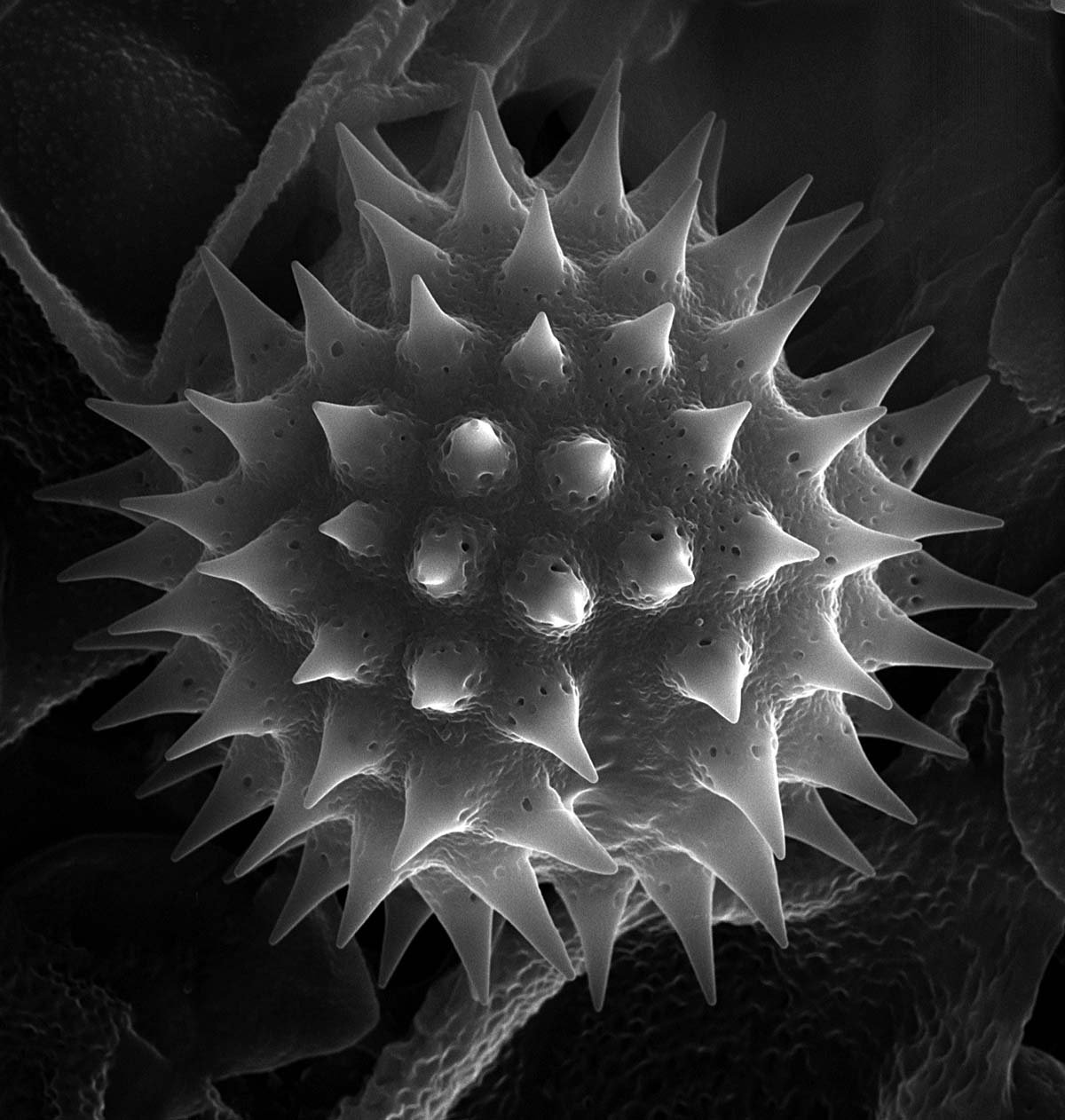This perfectly square grayscale image showcases a highly detailed, spiky sphere, reminiscent of a coronavirus cell seen under a high-powered electron microscope. The background is predominantly black with some faint light-gray, textured lines and blobs adding subtle depth. The central spiny sphere is composed of multiple layers of pointed tips, organized in increasing diameters from top to bottom. The tips, numbering approximately 50, exhibit varying shades from white at the edges to darker gray and black, emphasizing the sphere’s texture and elevation. This intricate, symmetrical structure appears to be part of or resting on a lesser-defined blob in the background, enhancing its prominence in the otherwise unembellished setting.